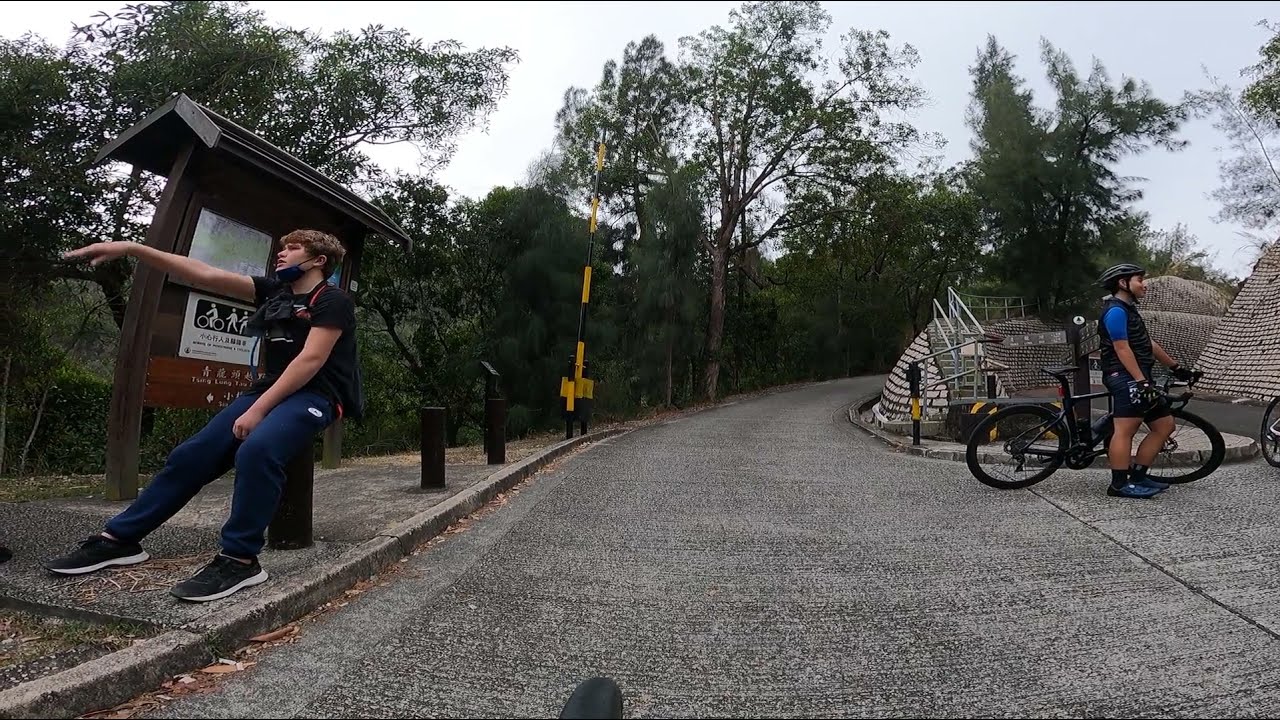The image depicts a narrow, uphill road that curves through a park intended for biking and hiking. On the left side, a man with brown hair, wearing a black shirt, blue sweatpants, a mask on his chin, and black and white shoes, sits on a black pillar beside the sidewalk. Behind him, there are two more black pillars, and a post board with a triangular roof, which features a poster and possibly provides information about the trail. On the right side of the image, another man stands next to a black bicycle. He is wearing a cycling uniform consisting of a black helmet, a blue short-sleeved shirt, a black vest, and black pants. Behind this man is a flight of stairs with a railing, leading uphill. The image background is filled with lush green trees, indicating the park-like setting. Overhead, the sky appears mostly white, likely due to overcast conditions or bright lighting.